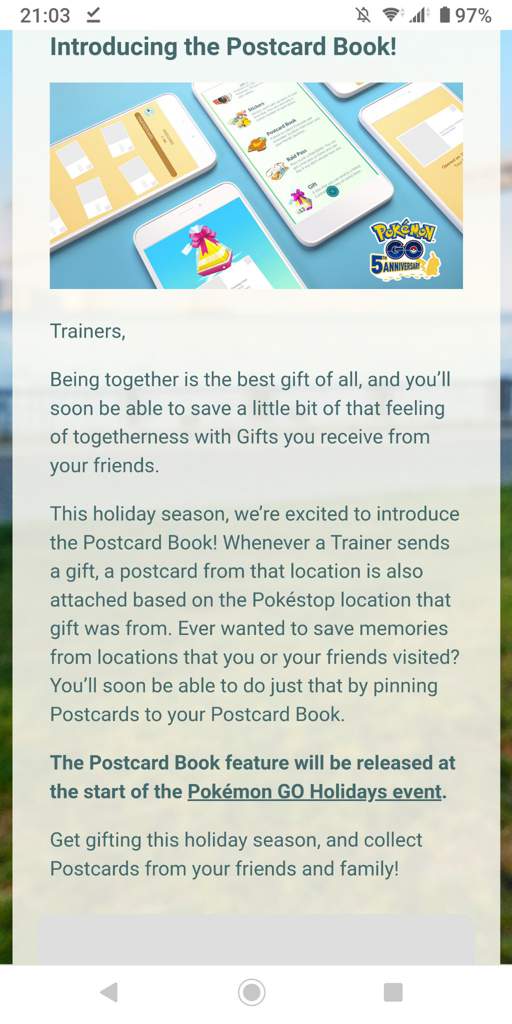This image captures a cell phone screen displaying a promotional announcement for a new feature in Pokémon Go. The phone’s status bar shows "2103" in the top left corner and includes icons for a wireless signal, cellular connection, and a battery at 97% in the top right corner. The headline reads, "Introducing the Postcard Book," followed by an image montage of several phone screens displaying different pictures. 

Below this, the text elaborates on the new feature: "Trainers, being together is the best gift of all and you'll soon be able to save a little bit of that feeling of togetherness with gifts you receive from your friends. This holiday season, we’re excited to introduce the Postcard Book. Whenever a trainer sends a gift, a postcard from that location is also attached based on the Pokéstop location that gift was from. Ever wanted to save memories from locations that you or your friends visited? You’ll soon be able to do just that by pinning postcards to your Postcard Book."

The announcement highlights in bold text, "The postcard book feature will be released at the start of the," with "Pokémon Go Holidays Event" underlined for emphasis. The message continues, "Get gifting this holiday season and collect postcards from your friends and family."

At the bottom of the screen, navigation icons are shown: a left-pointing arrow, a circle, and a square.